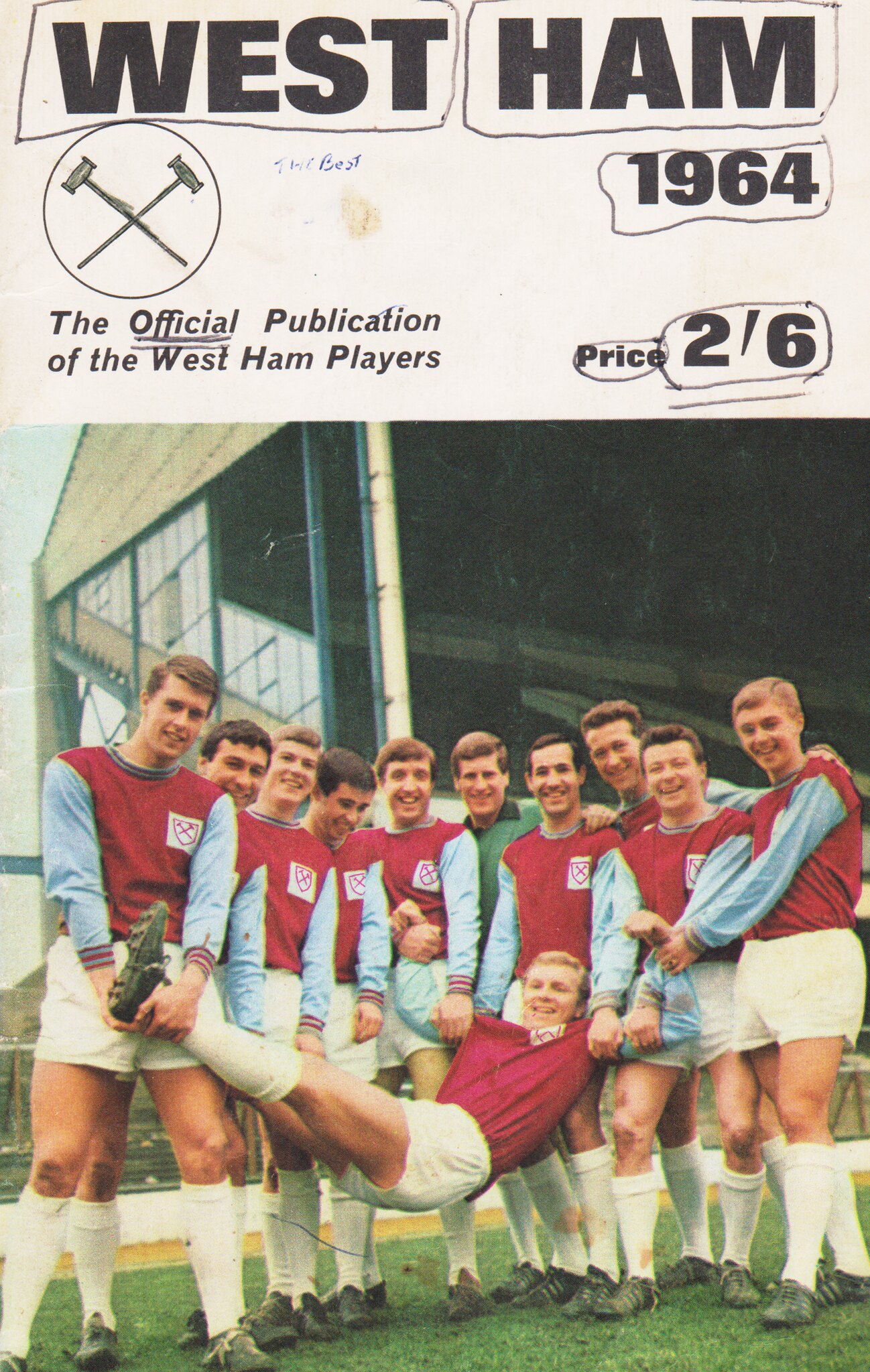This full-color brochure from 1964 is the official publication of the West Ham players, priced at two pounds six pence. The text, emphasized by a hand-underlined "official," marks its authenticity. Featured prominently on the brochure is a team photo taken outdoors in daylight, showcasing the players in their maroon shirts with blue sleeves, white shorts, and cleats. All the players, appearing to be young Caucasian males, are standing and smiling at the camera. Notably, one teammate is being whimsically held aloft, supported by his arms and legs, adding a playful touch to the scene. Despite its vintage appearance, the vibrant colors and joyful expressions capture the team's camaraderie and spirit.